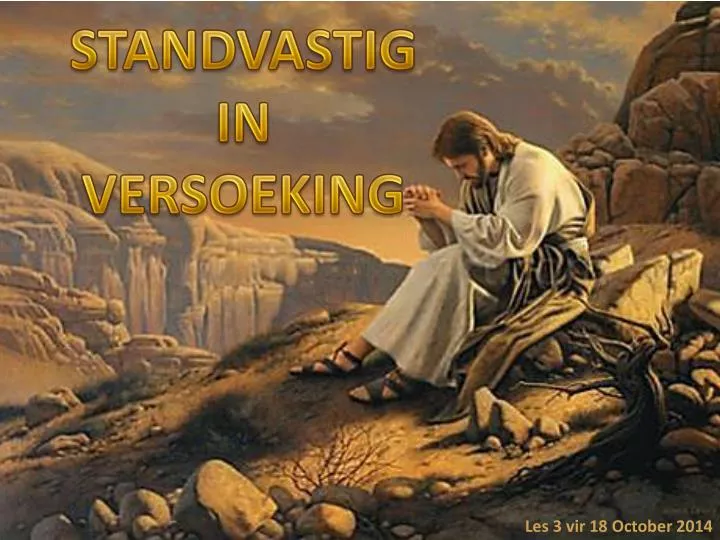The image depicts an artwork, possibly a card, featuring a man who resembles Jesus, seated slightly right of center on a rocky cliff. He is dressed in a white frock with a gray garment underneath, and he's wearing sandals. His head is bowed, and his hands are clasped in front of him, resting on his knees. The scene around him includes a small tree, several rocks, and a barren, tan dirt ground with some sparse, whispery weeds. The background showcases rugged, stone cliffs that rise on the right side of the image and extend across to the left, interspersed with some clouds and blue sky. The overall color palette includes hues of blue, white, tan, gray, brown, gold, yellow, and black, lending a somber, ancient atmosphere suggestive of biblical times. Text in large yellow letters on the top-left corner spells "Stan Vastig" and "Verso King," with additional text in smaller print at the bottom right reading "Les 3, Verner 18, October 2014." The man, likely Jesus, conveys a serene, contemplative mood in this historical and religious illustration.